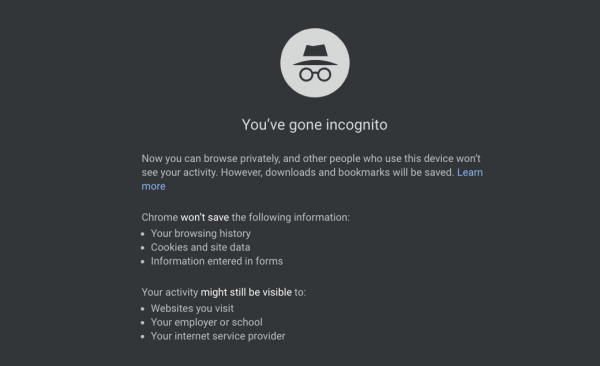The image depicts a webpage from the Chrome browser, specifically the Incognito mode landing page. At the top, a prominent circular icon on a white background features the outline of a hat and glasses in black, symbolizing private browsing. Accompanying text reads, "You've gone incognito," indicating that the user is now browsing in private mode. A message beneath elaborates that while users can browse privately and their activities won’t be visible to other users of the device, downloads and bookmarks will still be saved. 

Below this message, a blue "Learn More" button is displayed, signifying a clickable link for additional information. The text on the page further details that Chrome will not save browsing history, cookies and site data, or information entered in forms. However, it cautions that the user's activity might still be visible to the websites they visit, their employer or school, and their internet service provider.

The page's background is gray, and its text is primarily gray as well, except for the blue link. Key points, such as what information Chrome does not save and what may remain visible, are presented in bullet points for clarity. The layout also includes sections dedicated to custom settings and account details. Overall, the majority of the image is dominated by the gray background and white text, typical of Chrome's Incognito mode informational page.